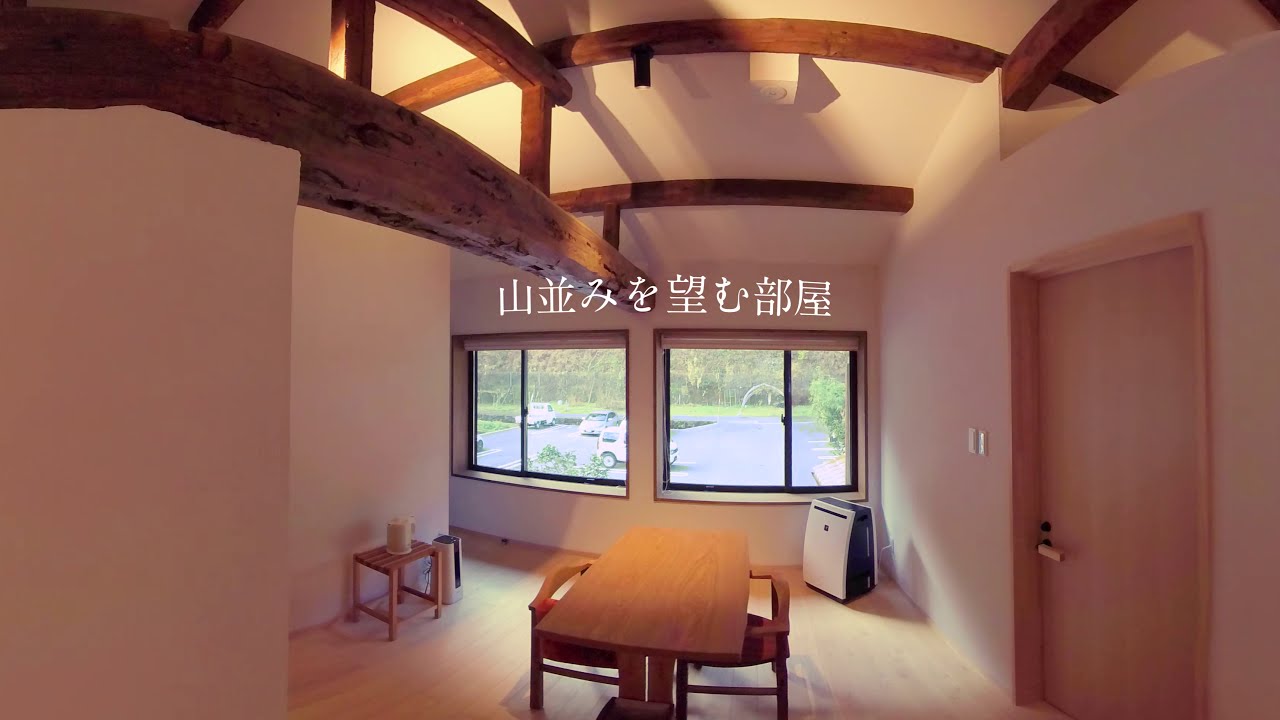The image depicts a room with white-beige walls and a light peach-colored wooden door situated on the right. The room features thick, dark brown wooden beams running along the ceiling. In the center, there is a rectangular wooden table with two matching wooden chairs. To the side, a small wooden side table is visible, topped with a white object and a pitcher. A small heater and white and black AC unit are also present in the room. The back wall has two large windows with black frames and blinds, revealing an outdoor parking lot with three or four parked cars and distant green trees and grass fields. Adding to the aesthetic, Asian characters overlay the image.